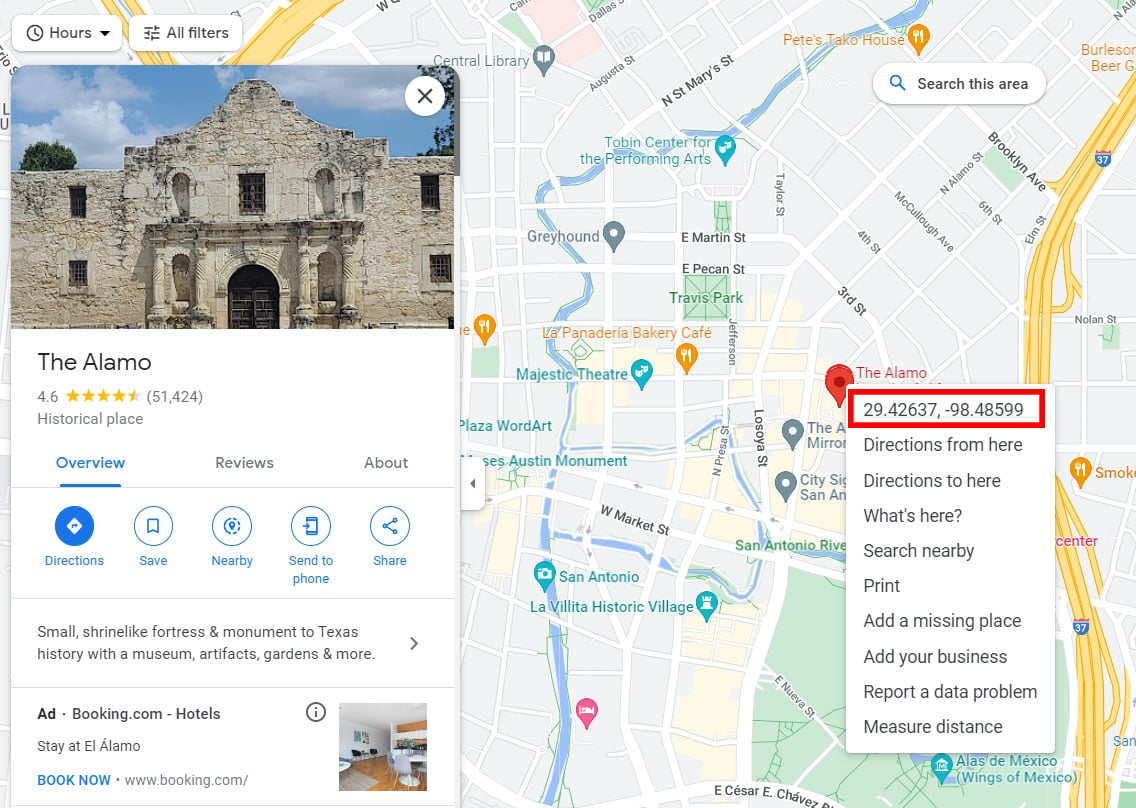The left-hand side of the map features a pop-up displaying detailed information about the Alamo. The map itself is color-coded with gray roads marked by white lines, while some streets, such as 4th Street, 3rd Street, Taylor Street, Brooklyn, and North Alamo, are labeled in black. Other notable roads include 6th Street, Elm Street, East Martin Street, and East Pecan Street.

The pop-up highlights a beige, ruin-like structure identified as the Alamo, situated under a sky dotted with blue and white clouds. The pop-up header reads "The Alamo," accompanied by a rating of 4.6 gray stars out of 5, based on 51,424 reviews. Labeled as a "historical place," the overview section is marked by blue, underlined text.

Additional navigation options include tabs for "Review" and "About," alongside five blue circles that offer options such as "Directions," "Save," "Nearby," "Send to Phone," and "Share." Below a thin gray line, the description reads: "Small shrine-like fortress and monument in Texas, noted for its historical significance. Features include a museum, artifacts, garden, and more."

An advertisement for Bookend.com hotels appears at the bottom of the pop-up.